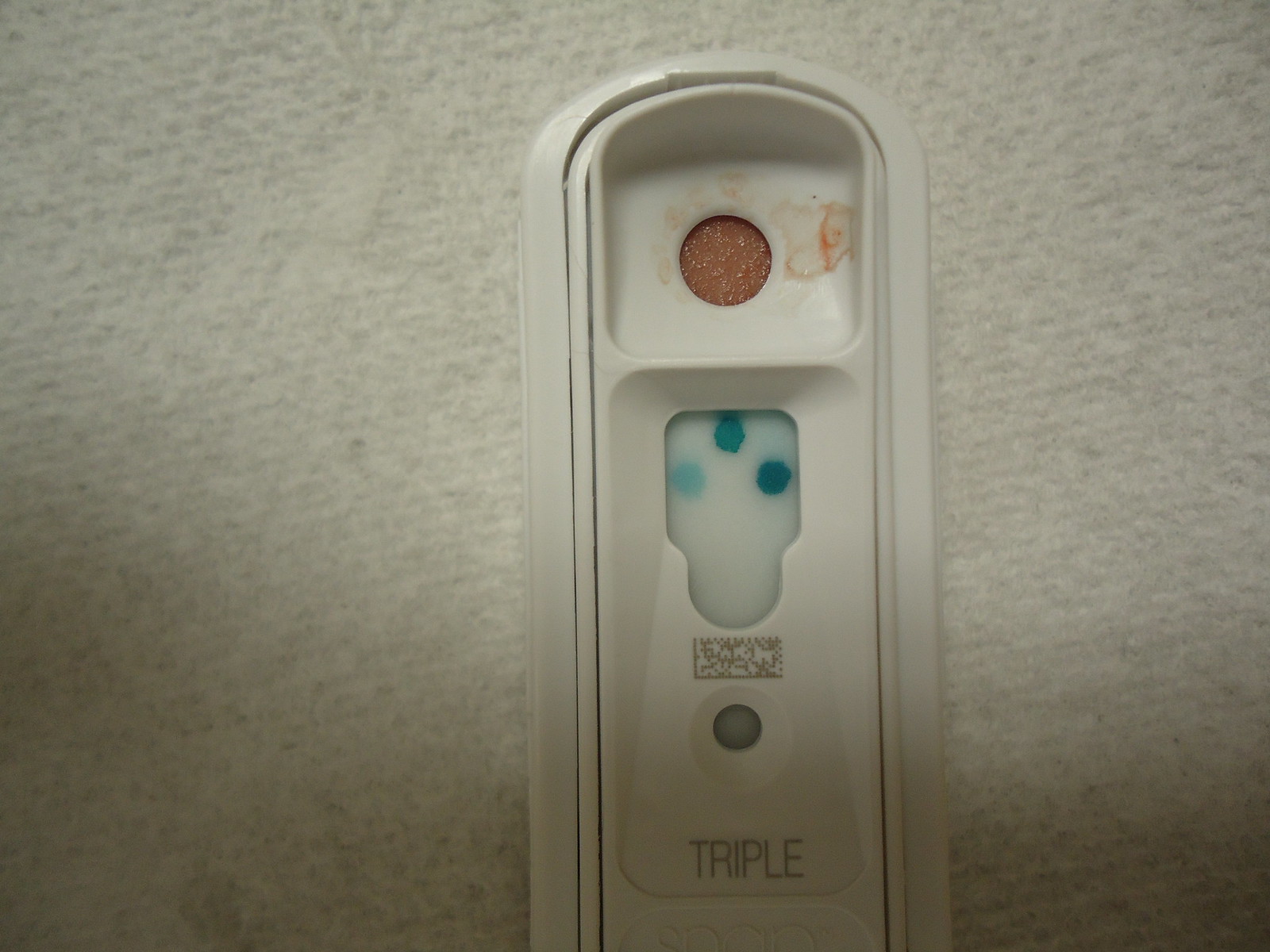In this image, a pregnancy test-like object is displayed on a white, partially translucent paper towel background, slightly off-center. The object has a long, rectangular shape with the bottom part cut off by the image frame and the top part curved with rounded edges. Made of white plastic, the object features an outer edge and an inner basin-like structure. Within this basin, there's a brown makeup-like substance with water stains around it, suggesting possible liquid exposure. Below this section, there's a shallower basin shaped like a square with a protruding circle, housing three blue dots—two in a darker bluish-green shade and one in a very light blue. Directly beneath the dots is a rectangular QR code, positioned above a small gray circle. At the bottom of the image, the word "TRIPLE" is prominently displayed in capitalized gray letters.